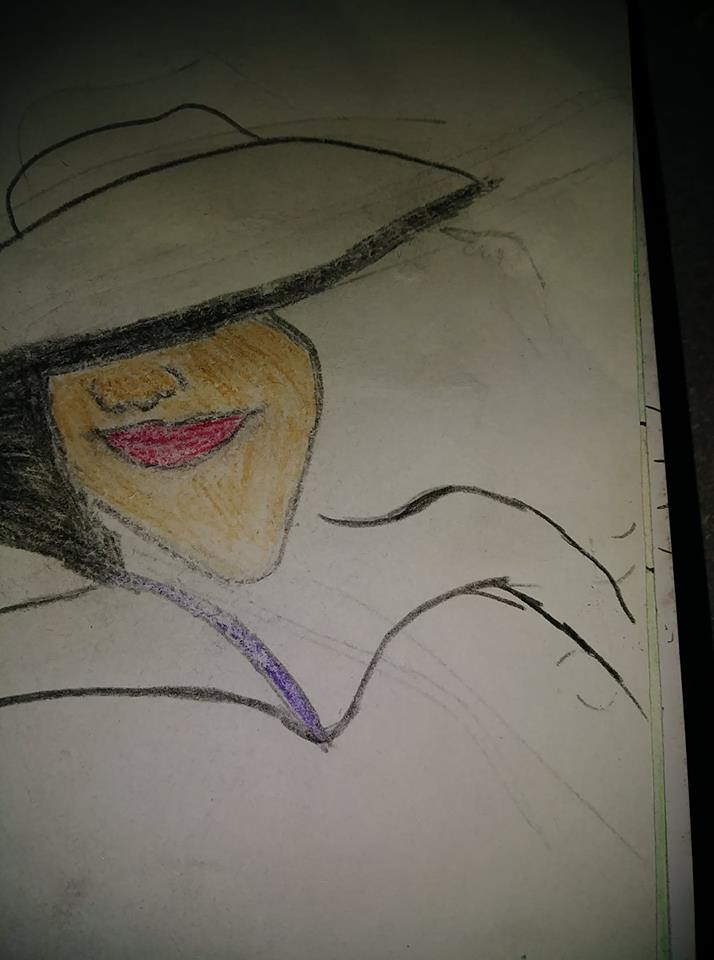This pencil and crayon portrait showcases a striking figure wearing a wide-brimmed hat that obscures the upper half of the face, covering the eyes and part of the nose. The hat's brim casts a shadow, adding an air of mystery to the character. Strands of hair peek out from the right side, suggesting the hair is swept to one side, while the left side remains hidden.

The face is meticulously outlined in black pencil, highlighting defined cheekbones and a pronounced, slightly pointed chin. The nose is broad, and the lips are full, colored vividly with red crayon and accentuated by black outlines. 

Moving down, the subject appears to be dressed in an off-the-shoulder or V-neck top, indicated by a curved V-shaped black outline. The shoulders are distinct, adding to the portrait’s sense of realism. The entire illustration seems to be set on drawing paper, laid flat on a table, emphasizing its hand-drawn nature and the textured quality of crayon and pencil. This image combines bold outlines with soft coloring, creating a unique and engaging visual experience.